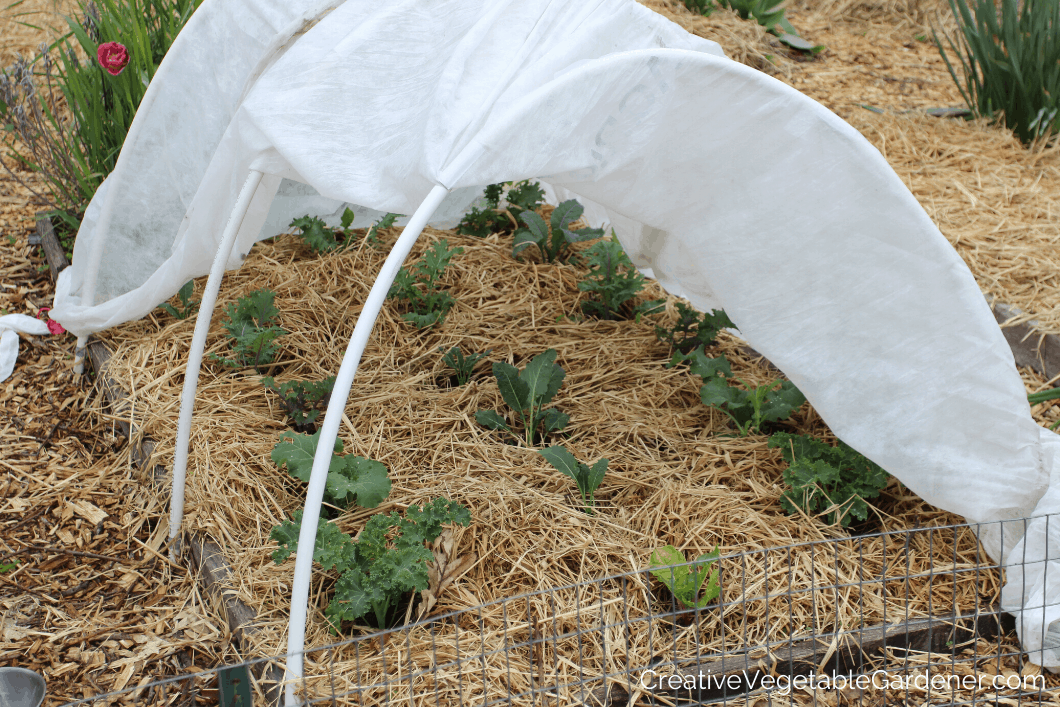The image depicts an outdoor scene featuring a homemade greenhouse. The structure is created using white arches draped with a white sheet that descends down the sides, likely to maintain warmth, similar to cheesecloth. The greenhouse covers a meticulously arranged garden bed, consisting of three rows of green vegetable tops protruding from a bed splayed with scattered hay. This temporary greenhouse setup sits in front of a backdrop of long grass, with a solitary red rose visible behind it. The garden bed is encircled by a short chicken wire fence, adding to its rustic charm. Across the bottom right corner of the image, there's a promotional banner reading "creativevegetablegardener.com," suggesting its use for advertising a website dedicated to vegetable gardening.